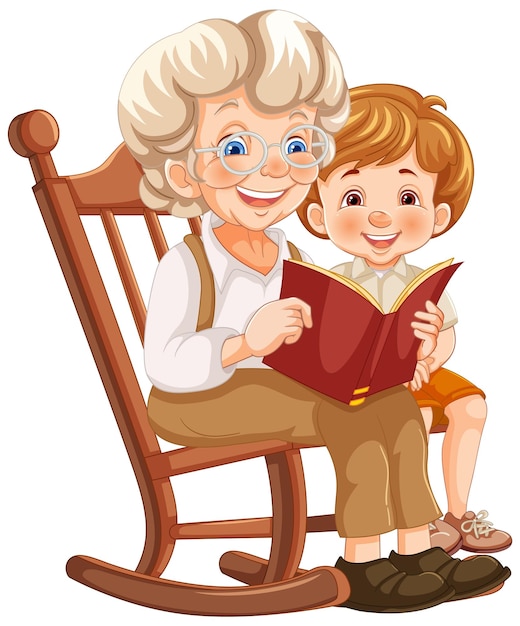This image is a light-hearted, cartoon-style illustration, possibly created with digital tools, that depicts a touching family scene between a grandmotherly figure and her grandson, both seated together on a brown wooden rocking chair. The grandmother, with her golden blonde, wheat-colored hair and matching eyebrows, has an animated and happy expression. She wears wire-framed glasses over her blue eyes and has a warm, welcoming smile that reveals her white teeth. Her attire includes brown suspenders over a white collared shirt, light brown pants, and dark brown shoes. The grandmother's nose and cheeks are tinged with pink, adding to her lively appearance. 

Sitting beside her is the young boy, her grandson, who shares the same cherubic cheeks and smiling expression. He has reddish, light brown hair and bright brown eyes. Dressed in a cream-colored collared shirt, orange shorts, and brown shoes, he looks well-put-together. Both characters appear deeply engaged and happy as the grandmother reads from an open book, sharing a moment of joy and connection. The detailed and clean rendering of their expressions, the clothing, and the setting highlights the affectionate bond between them, making the scene particularly heartwarming.